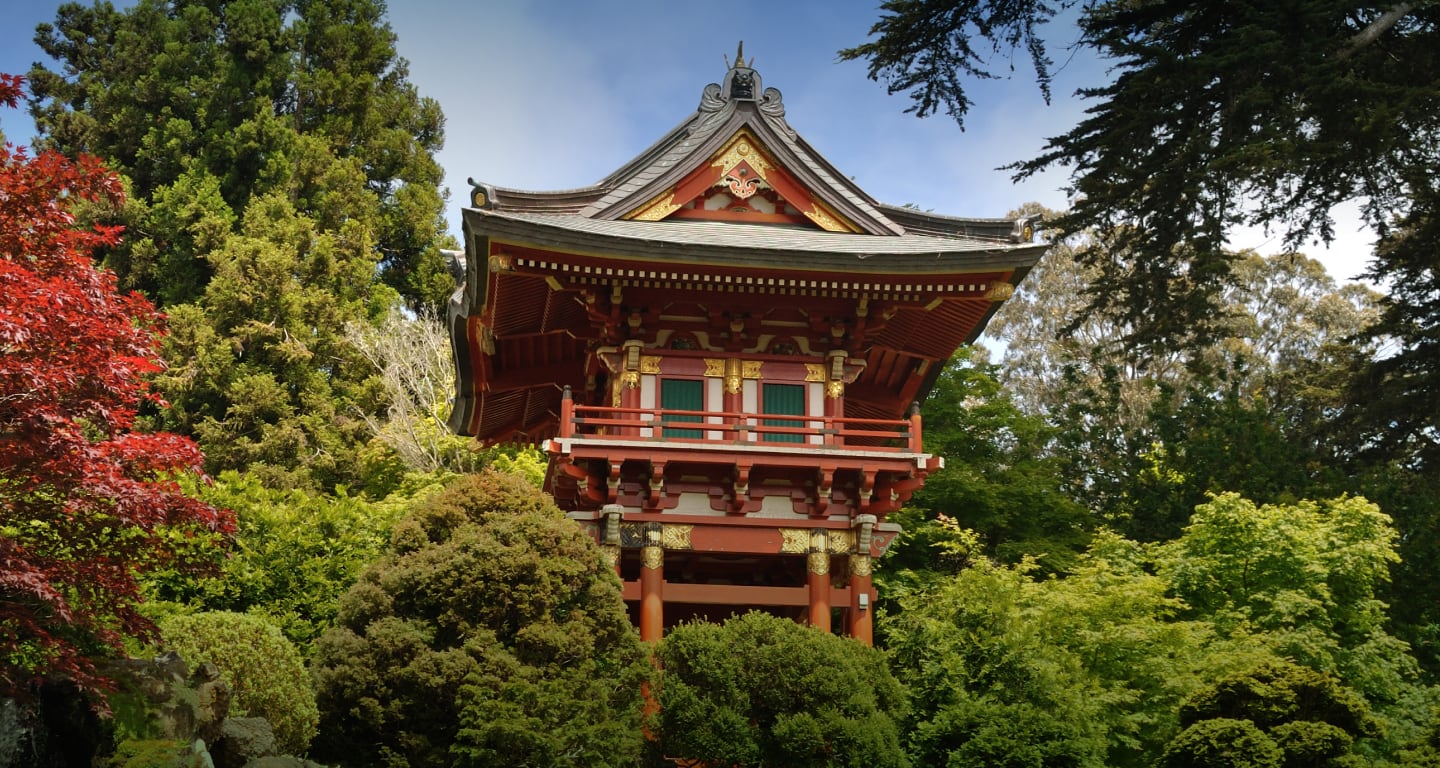This image depicts a serene Japanese tea garden under a blue sky dotted with wispy white clouds. The foreground and middle ground of the photograph showcase a stunning pagoda-style building, centered within the frame. This traditional East Asian structure is constructed with red-colored wood and accented with gold trim. The building is elevated on wooden circular posts with gold-capped tops. A flat wooden platform supports the structure at its base, leading up to a stone portion and another expansive wooden platform with supportive beams and a wooden railing. The roof of the pagoda is wider than the building itself, with gray shingles and intricate gray designs that provide ample protection from the elements. At the rooftop center, the structure peaks with a small Buddha figure embellishing the top.

The surroundings are lush with various trees and shrubs. On the left-hand side, a vivid Japanese maple with red and orange leaves, indicative of autumn, stands out. Coniferous trees occupy the upper left, bottom left, and upper right-hand corners, while tall deciduous trees frame the far distance on the back right. Dense green bushes surround the pagoda, adding layers of greenery. The right-hand side of the image is notably illuminated by sunlight, casting a warm glow across the serene landscape.